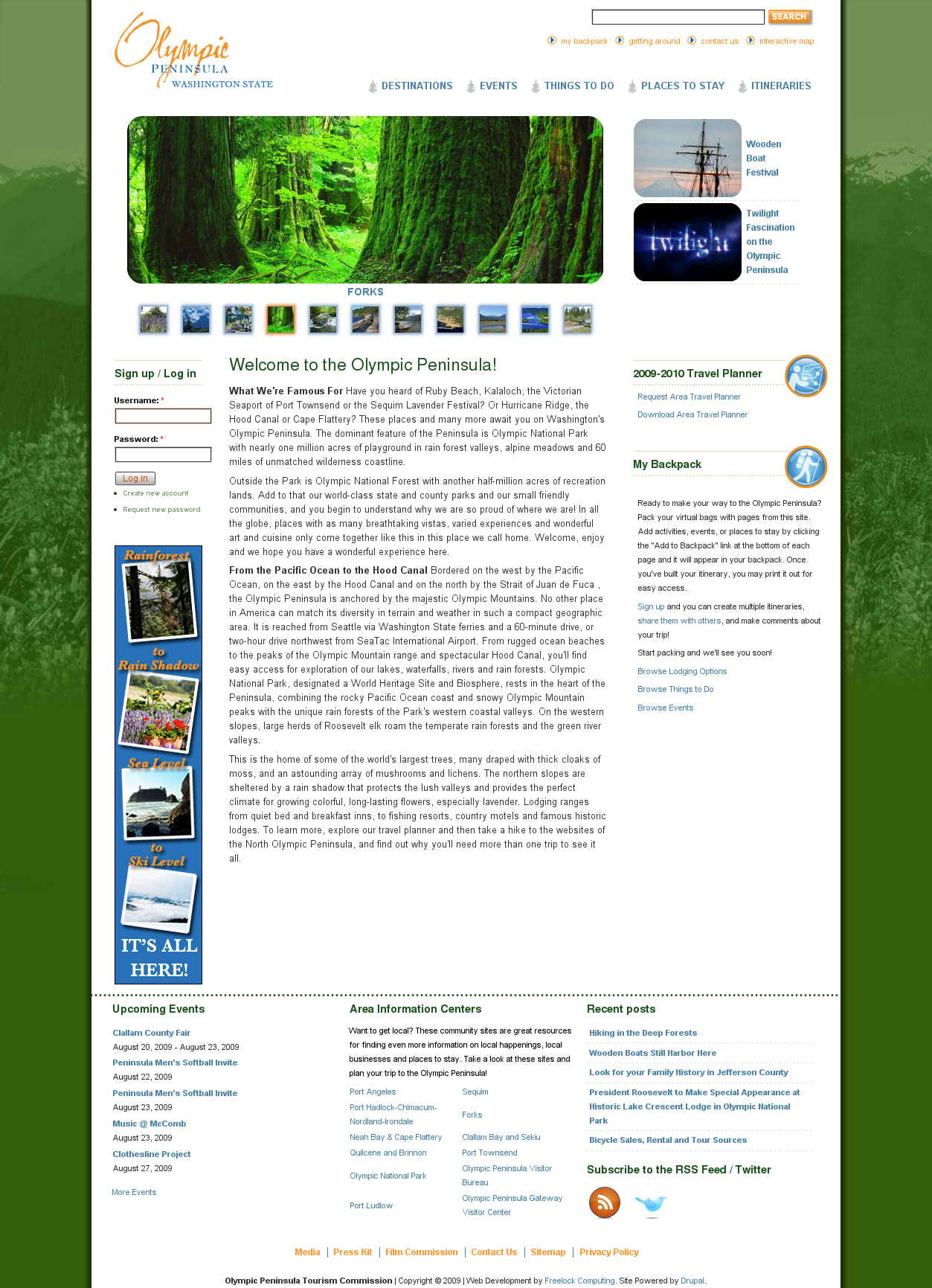Welcome to the Olympic Peninsula: Your Gateway to Natural Wonders and Adventure

The webpage for the Olympic Peninsula prominently features a comprehensive navigation bar at the top, including a search function and menu options such as "My Backpack," "Getting Around," "Contact Us," and an "Interactive Map," each accompanied by a play button-style icon indicating they are hyperlinks.

Directly beneath the header, the title "Olympic Peninsula, Washington State" is displayed prominently, with the word "Destinations" in blue, likely serving as another hyperlink. Further navigation options allow visitors to explore "Events," "Things to Do," "Places to Stay," and "Itineraries."

A detailed image carousel showcases key attractions. One featured event is the Wooden Boat Festival, highlighted with a picture of a sailboat, while another section emphasizes the area's "Twilight Fascination" with lush images of thick forest and colossal tree trunks.

The section below warmly welcomes visitors to the Olympic Peninsula, explaining the region's renowned spots like Ruby Beach and offering an overview from the Pacific Ocean to the Hood Canal. It provides an area for users to sign up or log in with a username and password, enhancing user experience and personalized interaction.

Additional visual content portrays diverse landscapes, including rainforests and sea level views. On the right-hand side, for more detailed planning, visitors can access a travel planner through clickable options to either request a physical copy or download a digital version.

The bottom of the webpage offers extensive information on upcoming events, key areas of interest, information centers, and recent posts, ensuring visitors are well-informed and inspired for their visit.